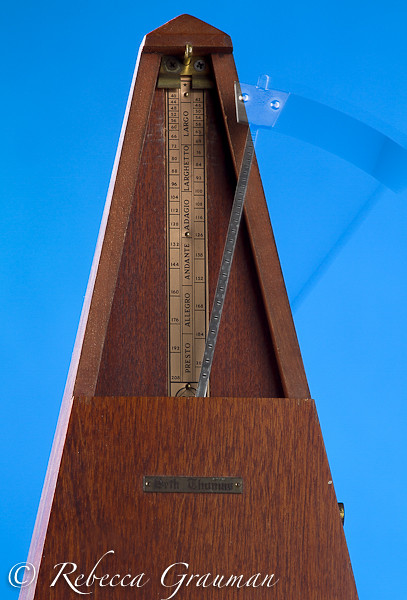This photograph showcases a classic wooden metronome set against a vibrant sky blue background. The metronome, with its characteristic triangular shape, features a partially covered exterior, with the wooden cover extending halfway up the body, leaving the upper portion exposed. A clear label reading "Seth Thomas" adorns the front, confirming the maker's name.

The exposed upper section of the metronome reveals a brass scale marked with various tempo indicators such as Presto, Allegro, Andante, and Adagio, guiding musicians through different speed settings. At the center of this section is the pendulum, also known as the wand, which traditionally swings back and forth to maintain a steady rhythm.

In this particular shot, the shadow of the pendulum is cleverly captured, illustrating its motion from the middle of the photograph to the far right. The shadow creates a sense of movement, visually representing the metronome's function of keeping time. The intricate details, from the brass scale to the polished wooden finish, are clearly visible, emphasizing the craftsmanship of this timeless musical tool. The photograph ingeniously combines stillness with an illusion of motion, encapsulating the essence of the metronome's rhythmic precision.